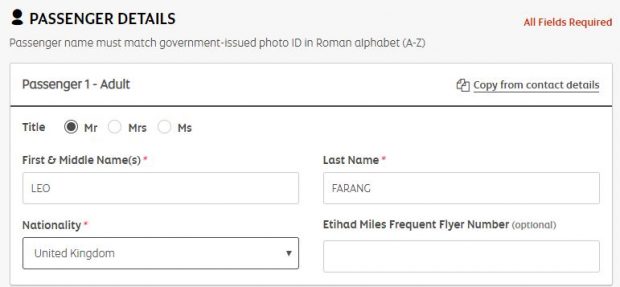This image is an edited and cropped screenshot capturing a segment of the passenger details section within an airline booking form. Dominating the top left of the section are the words "Passenger Details" in bold, large black letters. Beneath this, in smaller grey text, is the note: "Passenger name must match government issued photo ID in roman alphabet (A-Z)."

On the top right, there is a prominent reminder, "All Fields Required," highlighted in bold red font. Below this header, a large white rectangular section begins with the title "Passenger 1 - Adult" on the left. Adjacent to it on the right is an option labeled "Copy from contact details," paired with an icon of little papers with folded edges.

The form continues with a row starting at the far left labeled "Title," offering options such as Mr., Mrs., and Miss, with "Mr." currently selected. Subsequent fields organize passenger information input: text boxes for first and middle names, last name, and nationality.

At the bottom left, a dropdown box provides additional selection options, while the bottom right features a field labeled "Etihad Miles Frequent Flyer Number (Optional)."